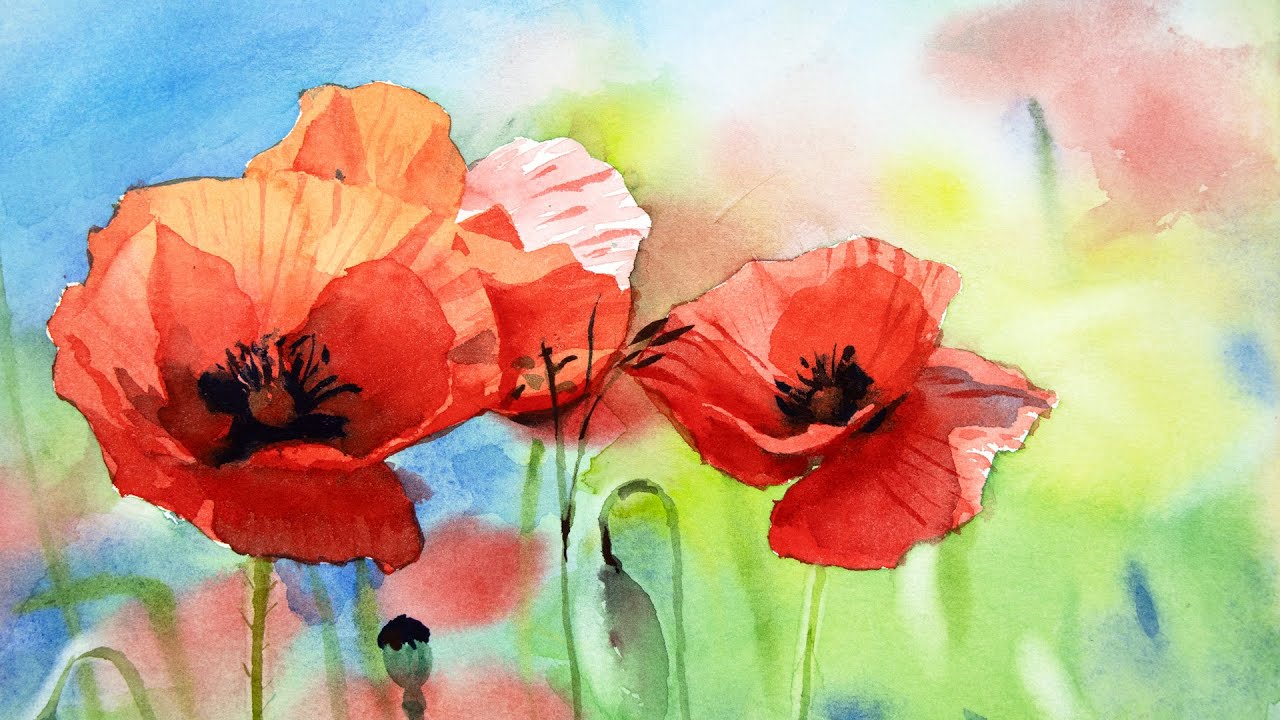This watercolor painting, rendered in pastel shades, features a rectangular composition wider than it is tall. Dominating the scene are red flowers with delicate accents of orange, pink, and white, their vibrant petals contrasted by dark-colored pistils at their centers. Green stems anchor the flowers, some culminating in unopened buds, particularly noticeable toward the left side. A couple of these buds appear to be wilting to the left, contributing to the image's transient beauty. The background is a harmonious blend of muted blues, greens, pinks, whites, yellows, and occasional reds, merging seamlessly in classic watercolor fashion. Notably, the painting captures intricate details such as fine hairs protruding from the stem of a flower in the left corner, adding depth to the delicate portrayal of nature.